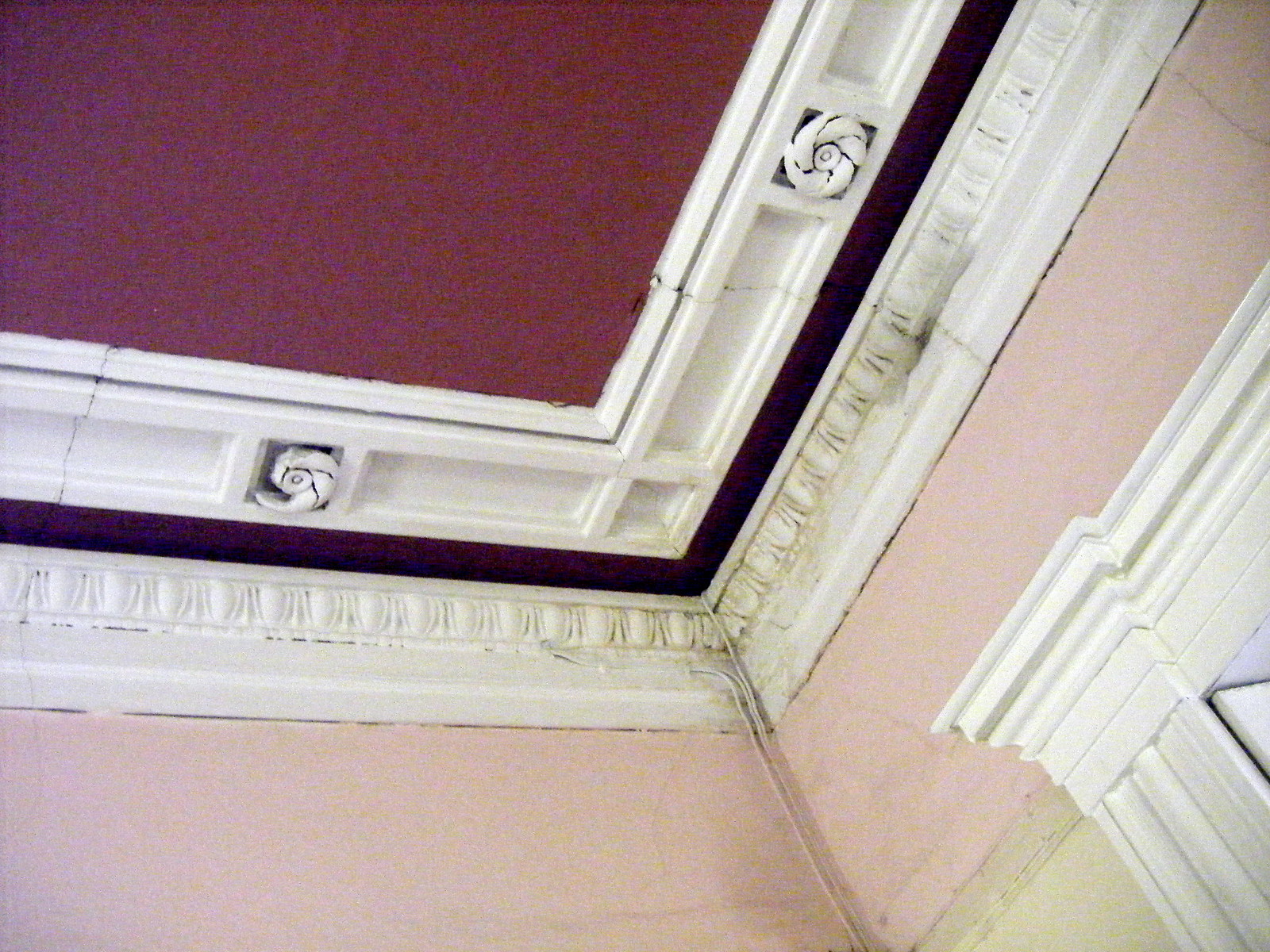In this image, we see the corner of a room that appears to be indoors, most likely inside a house. The ceiling is a dark maroon or burgundy color with white crown molding that runs along the edge where the ceiling meets the walls. The crown molding shows noticeable discoloration and stains, potentially mold, especially concentrated in the corners with a yellowish-green tint. The walls themselves display multiple colors: a soft pink hue dominates, while other sections appear tan. There is also a white beam extending across and down one side that seems slightly faded. Just visible in the bottom right corner is the archway of a door framed with white molding, which looks relatively clean compared to the rest of the room. The setting gives an impression of an older or possibly rundown building due to the crack and mold in the ceiling and discoloration on the walls.